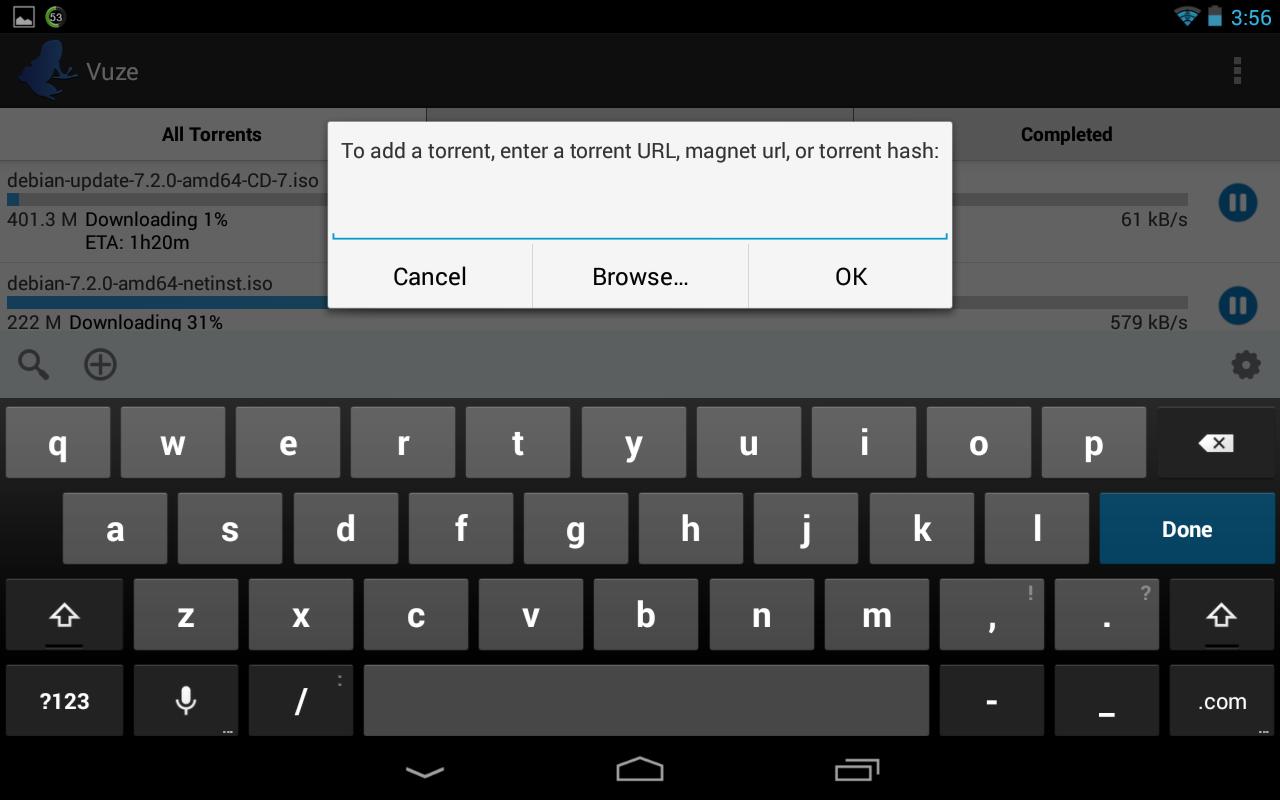The image shows a screen capture from a tablet or phone with a touchscreen interface. At the top left corner of the screen, the label "VUZE" is prominently displayed. The top right corner of the screen indicates that the device's battery is approximately half depleted and that it is connected via Bluetooth. The current time shown is 3:56. The main focus of the screen is a virtual keyboard, suggesting that the device is prompting for input. A pop-up window dominates the center, requesting the user to "Add a torrent," and provides options to enter a "Torrent URL," a "magnet URL," or a "torrent hash," with a noticeable difference in capitalization—the "Torrent URL" begins with capital letters while "magnet URL" is in lowercase. Below this prompt, there is a text field meant for entering the desired information, followed by three buttons labeled "Cancel," "Browse," and "OK." This indicates that the user is engaging in a torrent search and is being prompted to specify the type of torrent they wish to add.